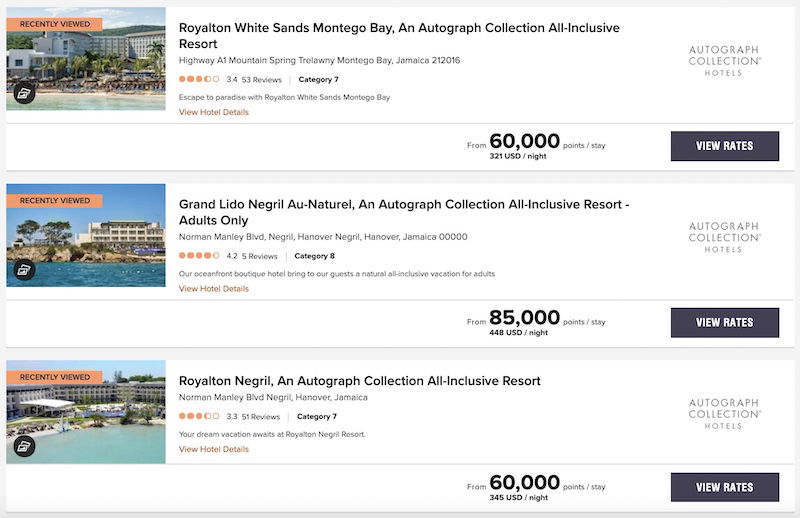The image showcases three rectangular boxes against a white background. Each box features a thumbnail image on the left depicting a hotel alongside a body of water. 

1. The top box is labeled with an orange strip stating "Recently Viewed" in the top left corner. The text reads "Royal White Sand Montego Bay, an Autograph Collection All-Inclusive Resort, Highway A1, Mountain Spring, Trailway, Montego Bay, Jamaica." Below this, it mentions the "Autograph Collection Hotel" priced at $60,000. Unfortunately, parts of the text are blurred and unreadable.

2. The middle box, also marked with the "Recently Viewed" orange strip, describes "Grand Lido Negril, an All-Natural Autograph Collection All-Inclusive Resort, Adults Only," with a price of $85,000.

3. The bottom box, similarly labeled with an orange "Recently Viewed" strip, details "Royalton Negril, an Autograph Collection All-Inclusive Resort," priced at $60,000.